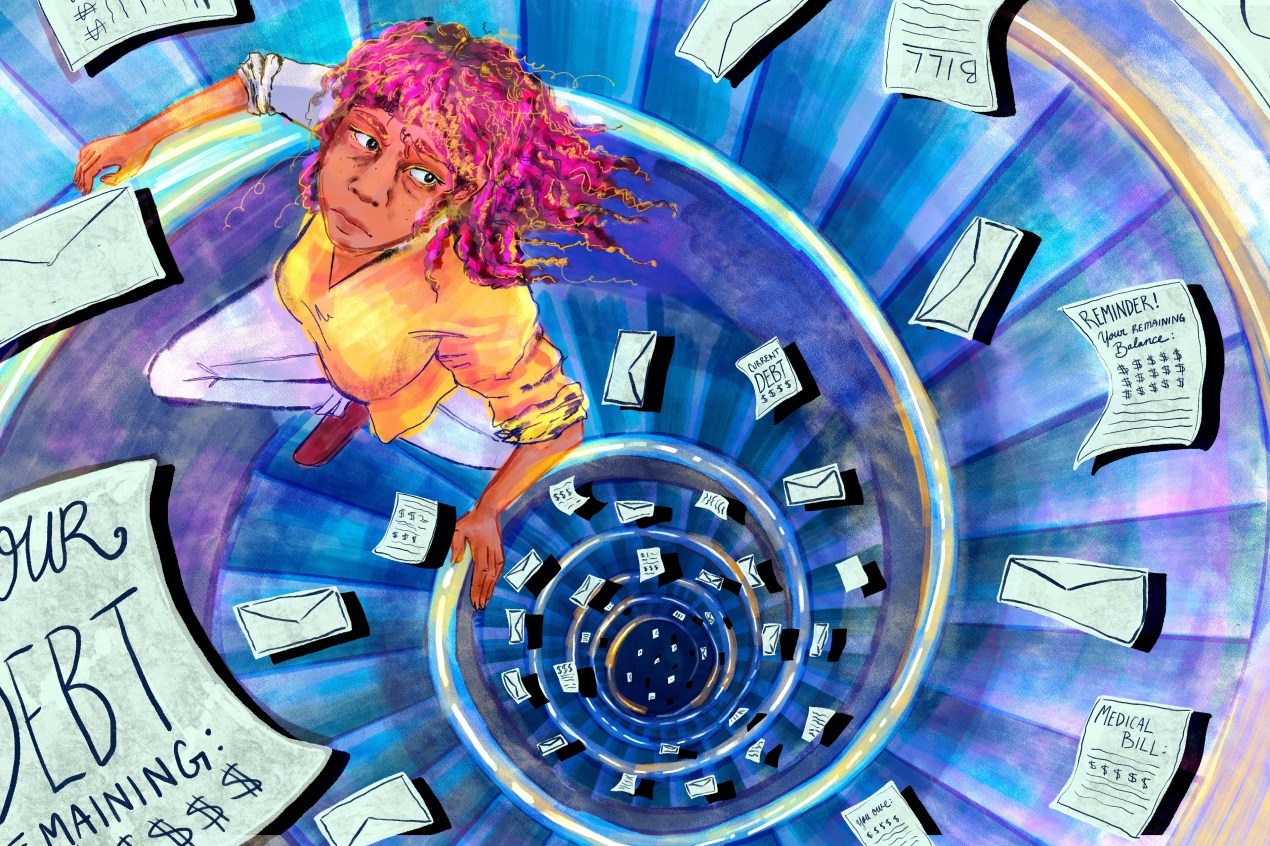This detailed artwork, rendered in a stylized, possibly watercolor medium, portrays a woman navigating an unending spiral staircase, symbolizing the relentless cycle of debt. Dominating the image is a distressed woman with wild purple hair, dressed in a yellow shirt, white pants, and brown shoes. Her expression is one of profound worry as she clutches the purple railing with a white handrail, ascending the blue stairs that seem to stretch infinitely. The staircase spirals upward from about six floors down, surrounded by a chaotic swirl of floating paper bills, each marked with ominous words like "Medical Bills," "Your Debt Remaining," and other financial reminders. The bright and cheerful colors starkly contrast the image's theme of suffering and desperation, capturing the endless and overwhelming nature of financial burden.